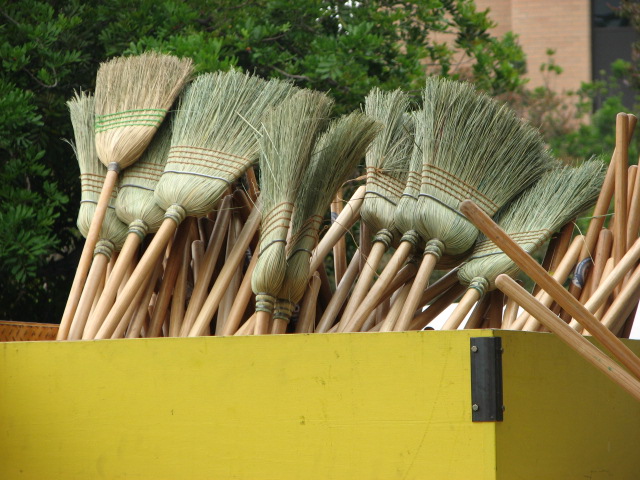This image depicts a large, yellow, open-topped wooden box filled with traditional handmade brooms. The box, which appears approximately 2-3 meters in length and about 1 meter wide, is reinforced with black metal pieces along the edges. The brooms inside are the old-fashioned type, featuring tan, corn bristle heads bound with blue and slightly orange-red thread at the base, and some have additional wrapping at the base where they attach to the wooden handles. The broom heads are arranged both up and down, with some showing the straw heads and others revealing the wooden poles. These brooms resemble the classic witches’ brooms with fanned-out bristles. The setting appears to be outdoors, possibly at a garden center or hardware store, as suggested by the presence of large, bushy-leaved trees and a glimpse of a light-colored brick building in the background.